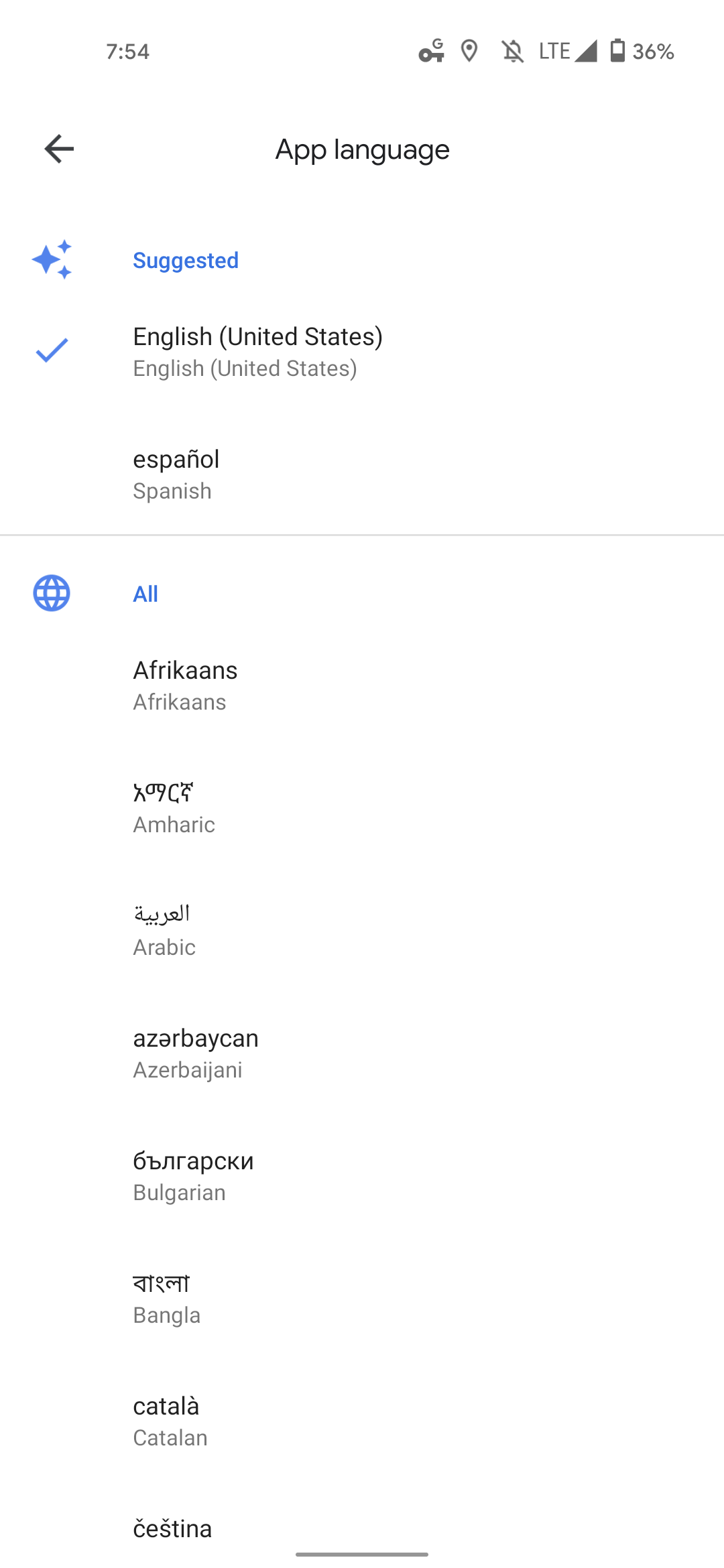The image captures a screenshot of an app's language selection screen at 7:54 AM, with full LTE signal and 36% battery remaining. 

At the top of the screen, an app language option field is displayed, labeled "App Language." Below, there are three blue stars to the left of the word "Suggested," which is also in blue. "English (United States)" is prominently displayed in black text, with a smaller gray text beneath it indicating the same language; this option is currently checked. Below it, "Español" (Spanish) is listed, both in English and gray text.

Further down, a thin separator bar divides the screen. Below it, a globe icon is followed by the word "All," indicating all available languages. The visible options before scrolling include:

- Afrikaans, listed twice
- Amharic, displayed as "Amharic" in blue with a symbol beside it
- Arabic, shown in Arabic script with "Arabic" in gray
- Azerbaijani, listed as "Azerbaijani" in English and another script
- Bulgarian, which appears in a script resembling Russian
- Bangla, resembling Hindi script
- Catalan, displayed as "Catalan"
- Cesky (Czech), partially visible, with its English translation obscured

Additionally, the screen includes interface icons such as a Google "G" with a key underneath, a map icon, and a bell icon indicating notifications are turned off.